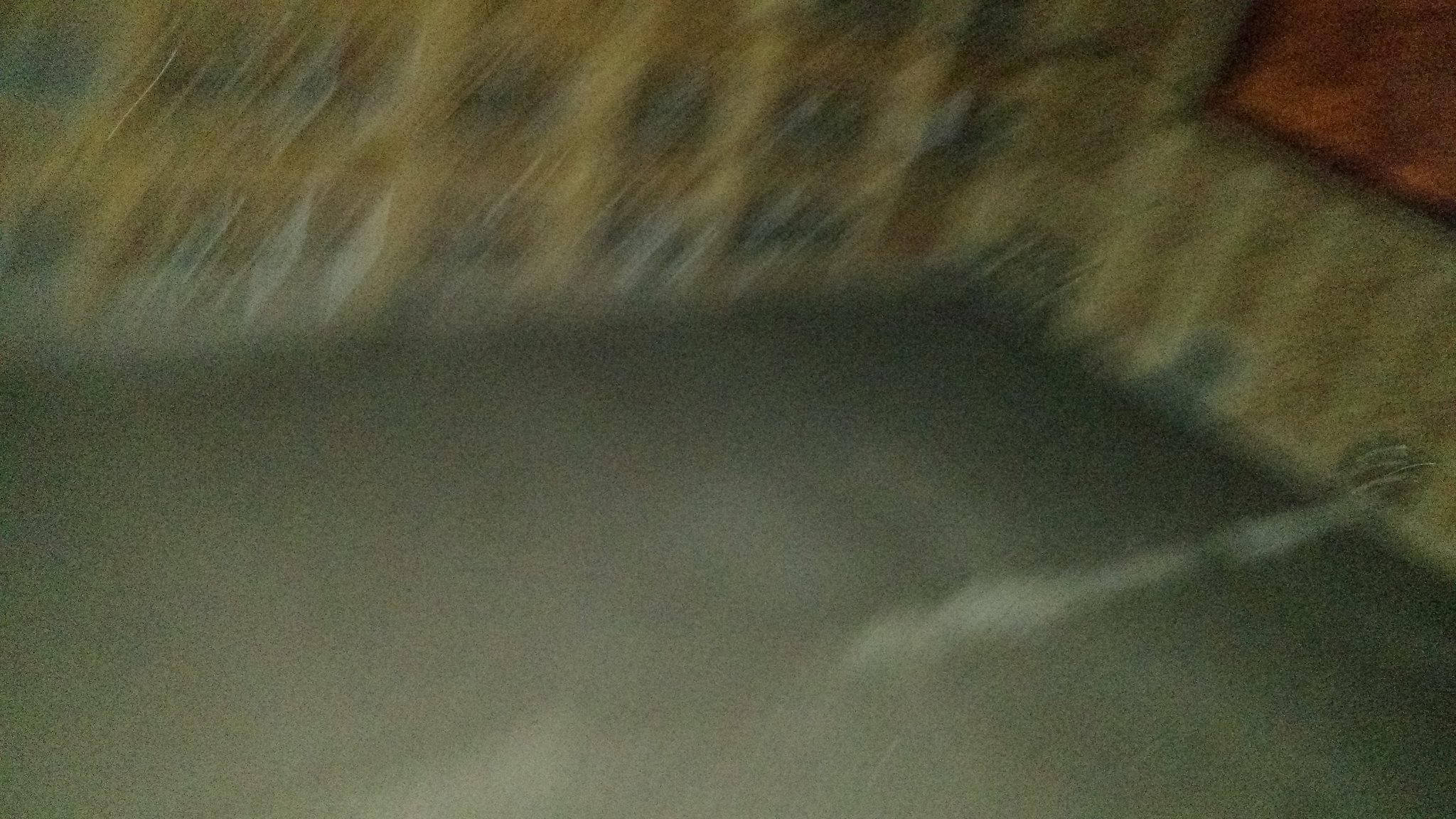A very blurry image reveals the early stages of construction within a room, featuring a concrete floor and walls framed out with 2x4s. In the upper right corner, a noticeable orange object can be seen amidst the framed wood and a partially constructed window. The entire scene appears distorted and partially obscured, as though viewed through a sheet of plastic. The concrete floor has several bright spots, likely illuminated by external light sources casting a glow across the surface.